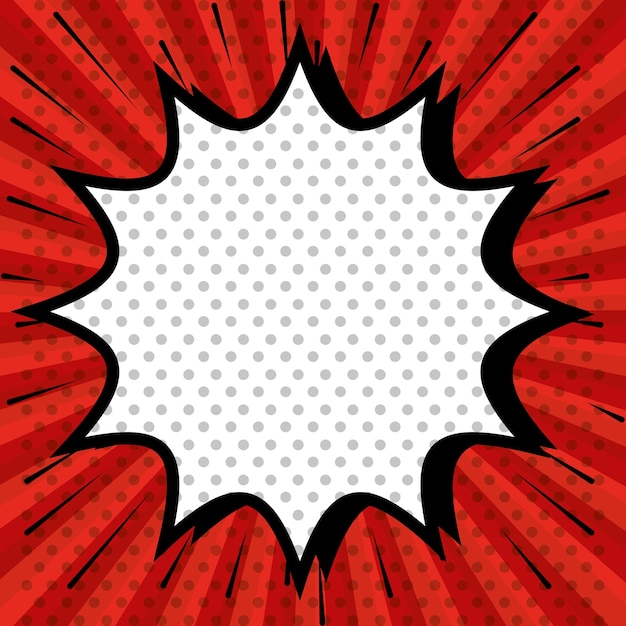The image depicts a vibrant, comic book-style explosion set against a deep red background adorned with various shades of red and dotted patterns. From the center of the explosion, jagged black lines radiate outward, enhancing the dynamic and action-packed feel reminiscent of classic comic book panels. The explosion's core is characterized by a prominent white starburst filled with light purple polka dots, and it is surrounded by additional white and grey dots. This dramatic focal point, structured with black outlines to accentuate its form and impact, is designed to evoke a sense of excitement and attention, akin to the dramatic "Bang!" or "Pow!" seen in superhero comics, especially during high-action moments like battles. The detailed interplay of colors and patterns emphasizes the importance and intensity of the depicted event, drawing viewers into the lively and energetic scene.